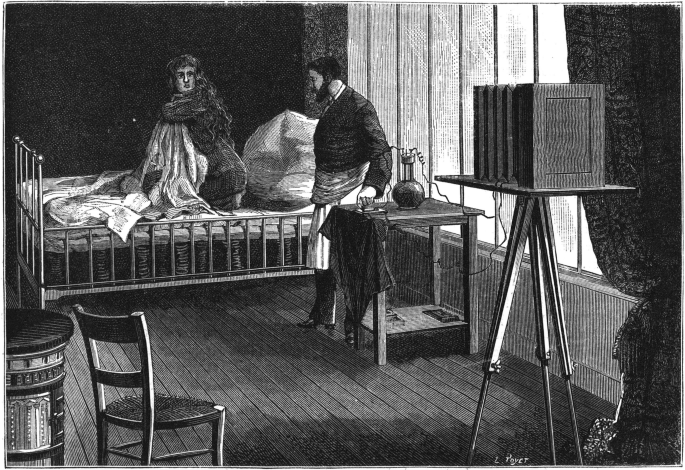In this vintage, black-and-white etching, a meticulously detailed room unfolds with a strong air of the past. On the right-hand side, a window draped in heavy brocade curtains filters light into the wooden-floored space. Centered is a brass bed with springs, occupied by a woman in a nightgown, her long hair cascading down her back. She clutches the light-colored sheets, gazing nervously towards a man nearby. This man, distinguishable by his beard and short hair, stands beside a table operating an electrical machine, reminiscent of a Tesla device, with a hand-held switch. On the right, a large, box-like old-school camera on a tripod is poised as if to take a photograph, with wires trailing from it. The detailed setting also includes various tables cluttered with objects such as a bottle and an end table, and a single wooden chair positioned in the lower right corner, completing the scene of this intriguing, staged photograph.